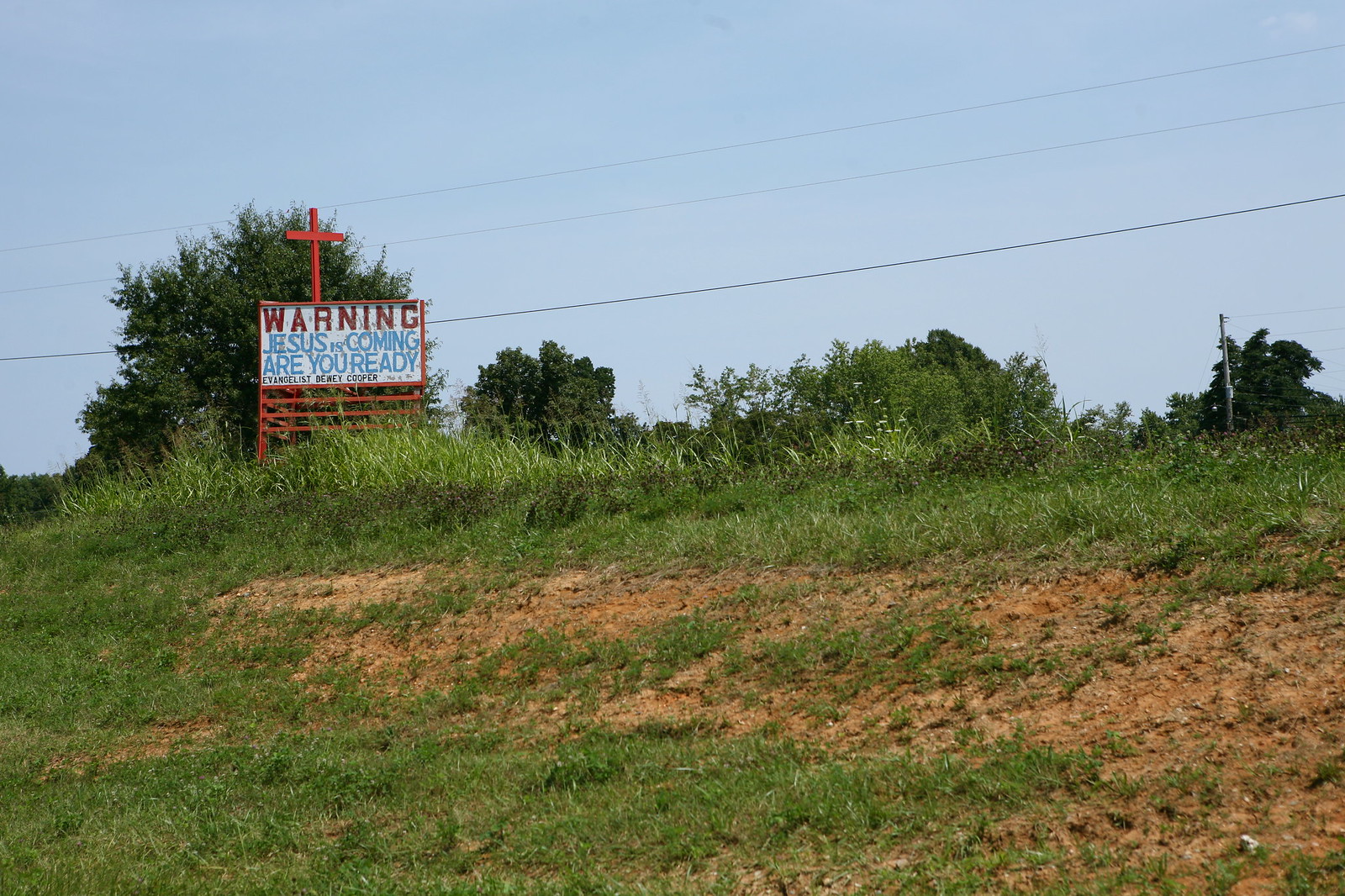The photograph captures a daytime scene of a patchy, rolling grassy hill with some exposed dirt. At the top left of the hill stands a prominent sign with a red frame and a red cross extending from the top. The sign features a white background with bold red text at the top reading "Warning," followed by blue text that states, "Jesus is coming. Are you ready?" Below this, in black text, it appears to credit Evangelist Dewey Cooper. To the left side of the hill, a large green bush is visible, and behind it, the image includes the tops of green trees and power lines stretching across a light blue sky.